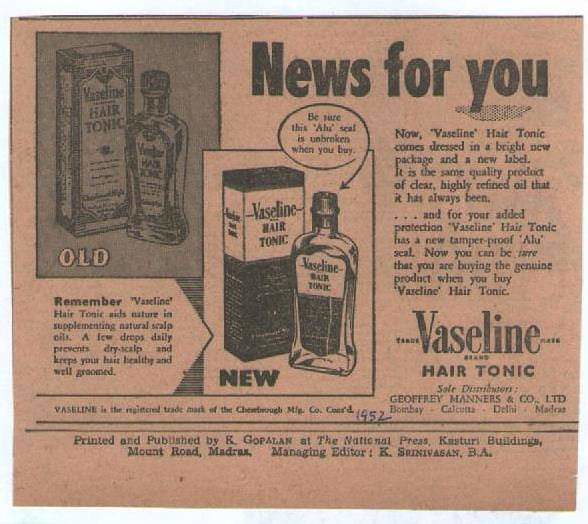This image is a detailed, aged newspaper clipping featuring an advertisement for Vaseline Hair Tonic, set against a background that has browned and faded over time, giving it a pinkish-brown hue. Dominating the top section is the headline "News for You." Below this, the ad contrasts the "old" and "new" packaging of Vaseline Hair Tonic, with a prominent illustration of both the old box and bottle on the left and the new on the right. 

Beneath the "old" label, the text reads: "Vaseline Hair Tonic aids nature in supplementing natural scalp oils. A few drops daily prevents dry scalp and keeps your hair healthy and well-groomed," with an arrow featuring a black outline pointing towards the "new" label. 

Nearby, another arrow within a circle makes the statement, "Be sure the seal is unbroken when you buy," stressing the importance of a tamper-proof seal. The "new" packaging also has an accompanying description that reads, "Now Vaseline Hair Tonic comes dressed in a bright new package and new label. It is the same quality product..." Despite some blurriness, the text continues to highlight the improved tamper-proof seal for added consumer protection, confirmed by the concluding reassurance that purchasing Vaseline Hair Tonic ensures the genuine product.

At the bottom of the advertisement, there is fine print stating, "Printed and published by K. Gopalan at the National Press, Kasturi Buildings, Mount Road." Additional minor text and lines are partially legible, suggesting publication details from 1952. The vintage ad, reminiscent of an era long past, provides an intriguing glimpse into historical marketing approaches.